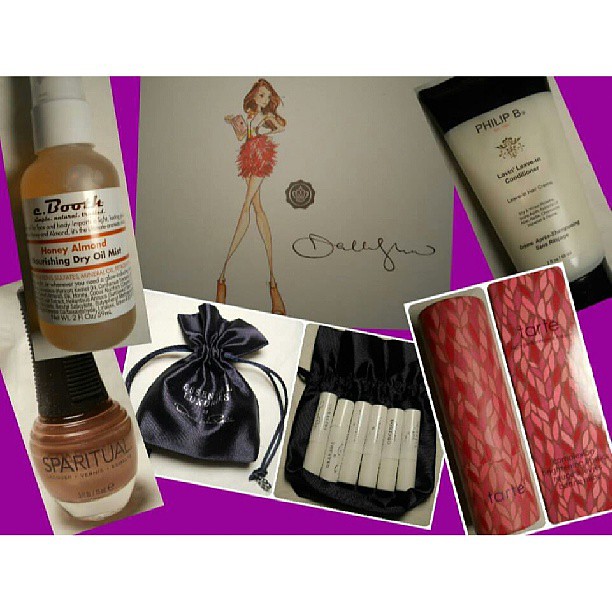In the image, we see a curated collection of beauty products presented in a way that resembles a collage set against a purple background. Central to the visual composition is a hand-drawn illustration of a stylish girl with long brunette hair, wearing a white top and a fuzzy pink skirt. Around this drawing are images of various beauty items meticulously arranged.

On the left side, there's a bottle labeled "Honey Almond Nourishing Dry Oil Mist." Below it, somewhat obscured, is a tan, cone-shaped bottle with a black cap labeled "Sparitual." Nearby, there is a black satin bag with silver text, which holds several small white canisters, resembling chapsticks or mini vials.

To the right, a red tube with the inscription "T-A-R-T-E" is visible, along with a cream bottle that has a black cap and "Philip B" written on it. Additionally, there is an ivory-colored bottle, presumed to be a conditioner, and a bottle of nail polish in a rusty red or orange hue.

The lid of the box housing these items appears to feature professional photos or cut-out images of the products, giving the presentation a scrapbook-like feel.